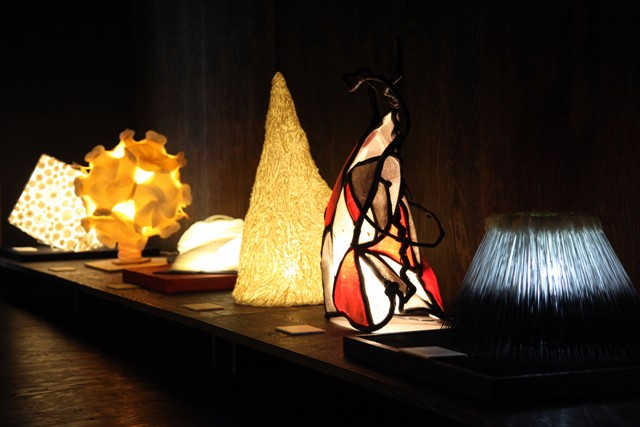The image depicts the top of a wooden table set against a matching wooden floor, both with a dark, brown hue. The table features an eclectic collection of six distinct objects, predominantly lamps and light fixtures, each with unique designs and illumination. 

To the left, there is a traditional blue lampshade, exuding a classic charm. Next to it is an elegant lampshade resembling stained glass, showcasing intricate, colorful patterns. A cone-shaped item, reminiscent of an upside-down gnome's hat, adds a whimsical touch to the arrangement. 

Among the other illuminated pieces, one is a vivid cube with a glowing light inside, reminiscent of a tesseract from popular culture, casting a warm, yellow hue. Beside it is a spherical object with a complex, spiked appearance, somewhat golden and evocative of a biological cell viewed under a microscope. Another peculiar item, difficult to discern, appears as a smudge, perhaps due to motion or focus in the photograph.

Completing the scene, a unique piece designed to look like a woman in a red, black, and white dress with her back turned is also noticeable. This mix of artistic, traditional, and abstract forms creates a visually captivating and diverse tableau of lighting fixtures.